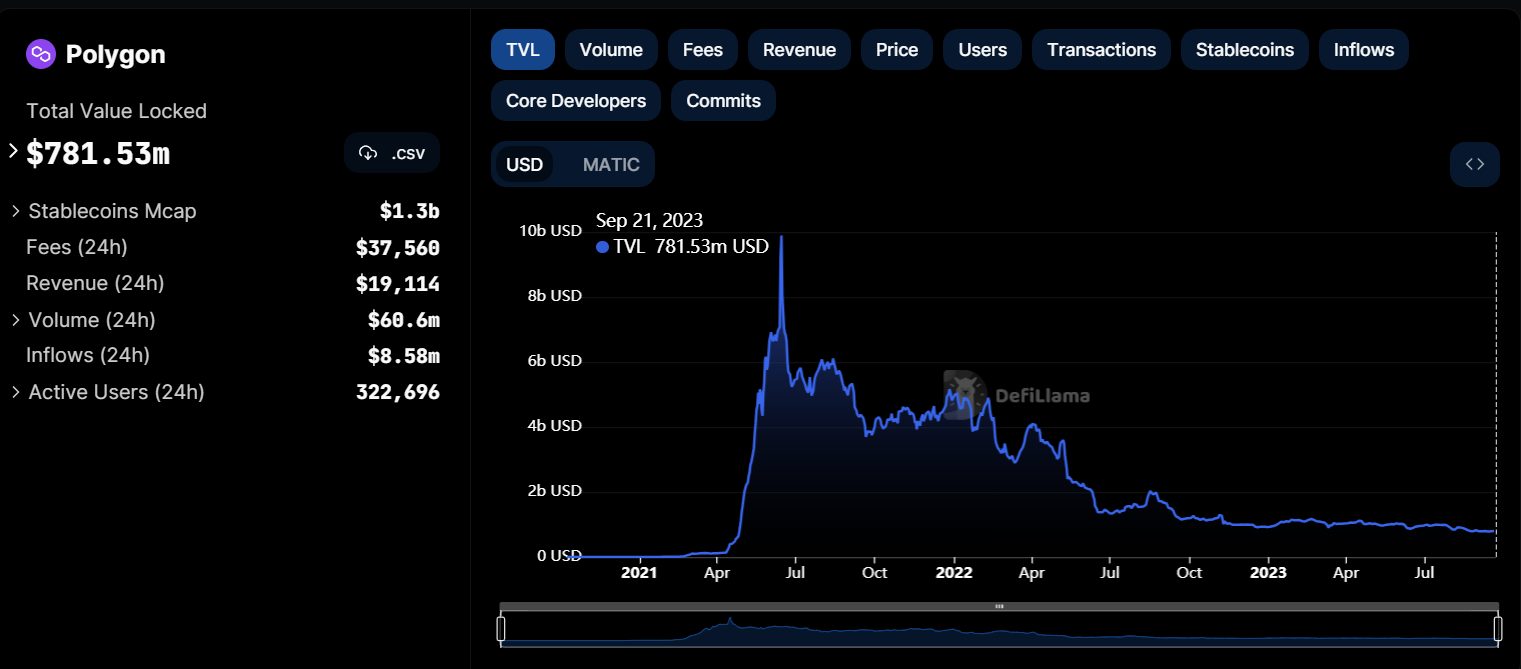A comprehensive chart displaying financial data related to a cryptocurrency or stock, likely Polygon, is presented in a sleek dark mode style with a black background. In the upper left corner, a purple circular logo featuring an infinity sign and the word "Polygon" in white is prominently displayed. The chart details various key metrics, including:

- Total Value Locked (TVL): $781.53 million
- Stable Coins Market Cap (MCAP): $1.3 billion
- Fees (24 hours): $37,560
- Revenue (24 hours): $19,114
- Volume (24 hours): $60.6 million
- Inflows (24 hours): $8.58 million
- Active Users: 322,696

The chart tracks various indicators such as TVL, volume, fees, revenue, price, users, transactions, stable coins, inflows, core developers, and commits. Display options include USD and MATIC, with USD currently selected.

The vertical axis ranges from 0 to 10 billion in 2 billion increments, while the horizontal timeline starts from 2021, marked with April, July, and October intervals through 2022 and 2023. A notable sharp spike is observed between April and July of 2021, with a subsequent gradual decline.

This chart offers a detailed, visual representation of Polygon's financial metrics and performance over the given period, providing insights into its market activity and user engagement.